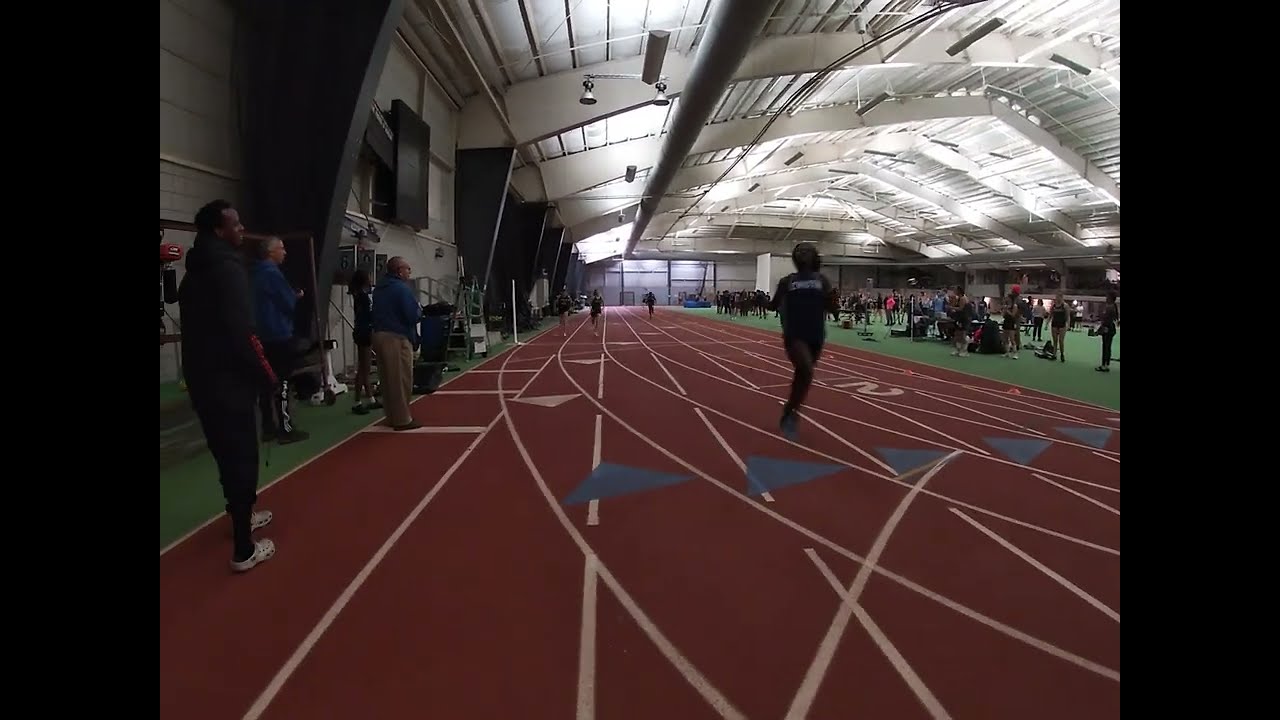This image captures an indoor track and field meet, focusing on a section of the 400-meter track as it curves around. The track, which takes up the center of the image, is brown or clay-colored with white stripes and includes directional arrows and the number two chalked on it. The setting is clearly indoors, featuring an enclosed structure with a roof and glass windows. Overhead, a domed ceiling houses numerous lights that illuminate the green astroturf inside the track. The track itself appears dimly lit by comparison. Off to the left, several people are standing and watching the event, while other individuals are actively running on the track. A clock is visible on the side wall, contributing to the detailed indoor setting. The colors evident in the image include green, white, brown, black, blue, dark gray, orange, pink, and gray. No text is visible anywhere in the image.